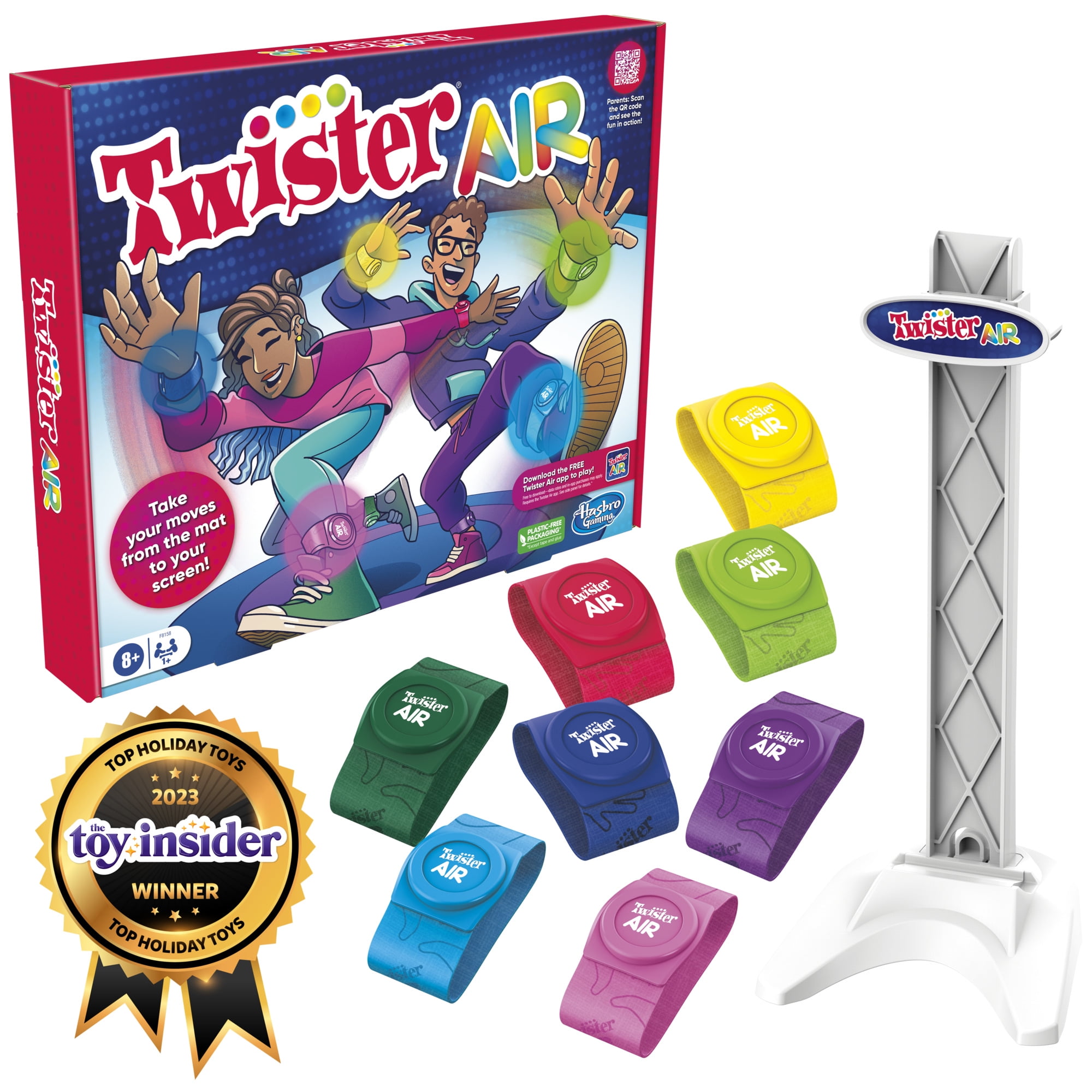This detailed image showcases an advertisement for the toy "Twister Air." In the top left corner, the Twister Air box prominently displays the product name against a primarily blue background, accented by red and multicolored text. The box features vibrant graphics of two players—a woman on the left and a man on the right—engaged in a game, both smiling and depicted in mid-action with one foot in the air. Each player is adorned with colorful glowing bracelets tied around their wrists and ankles, with hues ranging from purple and blue to various shades of green, yellow, pink, and red. Below the box, there is a golden pin sash award printed onto the white backdrop, which reads, "Top Holiday Toys 2023, The Toy Insider Winner."

To the right of the award, the individual Twister Air devices are neatly arranged. These include the brightly colored bands that players wear and a white plastic stand with a gray stem, also labeled "Twister Air," which presumably serves as storage for the bands when not in use. The entire setup emphasizes the interactive and colorful nature of the game, designed to take player's moves from the mat to the screen, making it evident why Twister Air has been recognized as a top holiday toy for 2023.